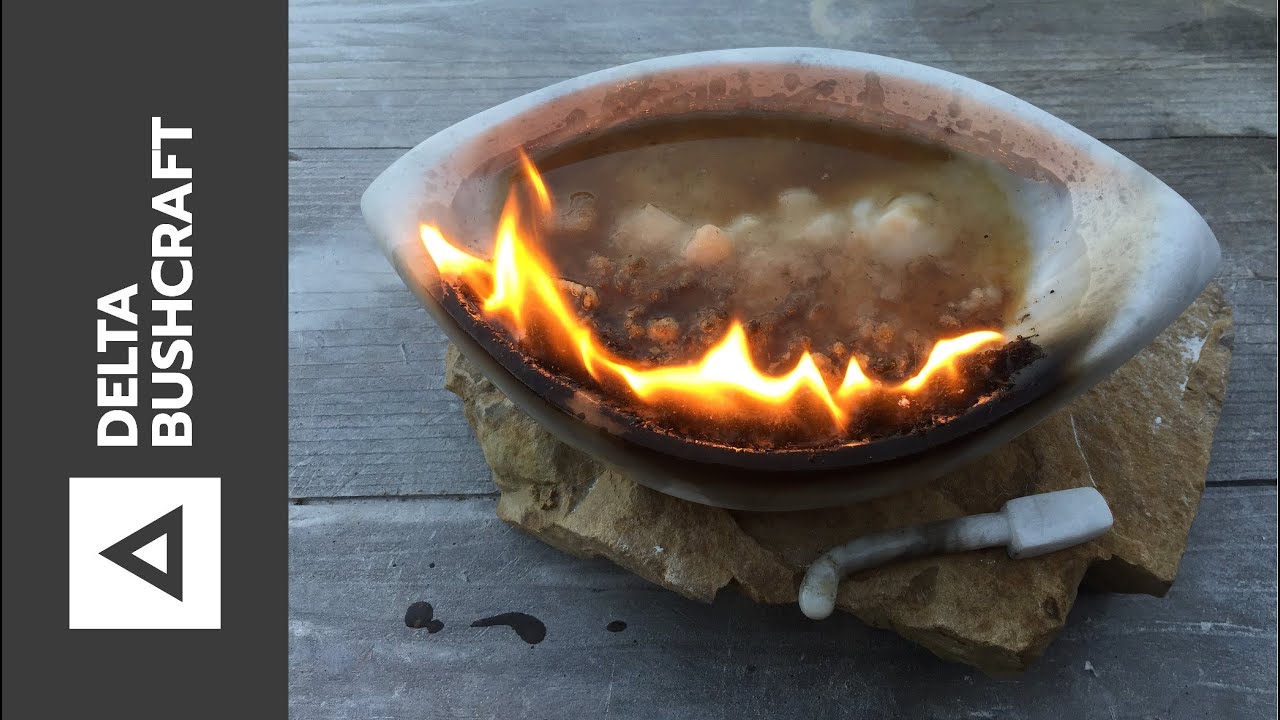In this detailed photograph presented as an advertisement, the centerpiece is an elliptical-shaped bowl, crafted from what appears to be a conch shell, featuring an intriguing combination of elements. The bowl is filled with a liquid, seemingly a brownish tone with white stones rising from it, and its edge is dramatically lit with vibrant orange and yellow flames. The bowl is centrally placed atop a flat, brown stone. Below the bowl, there's a distinct, white, hook-shaped tool resting on the rock. The setup lies on three horizontal planks of gray wood, creating a rustic backdrop.

On the bottom left of the image, a logo is prominently featured— a white square containing a gray triangle, which in turn encloses a smaller white triangle. Above this logo, the text “Delta Bushcraft” is visible in two rows of white print, reinforcing the branding. The overall composition, with its diverse array of colors including yellow, orange, black, white, gray, and brown, evokes a rugged, bushcraft-style aesthetic, suitable for outdoor or survival gear promotion.